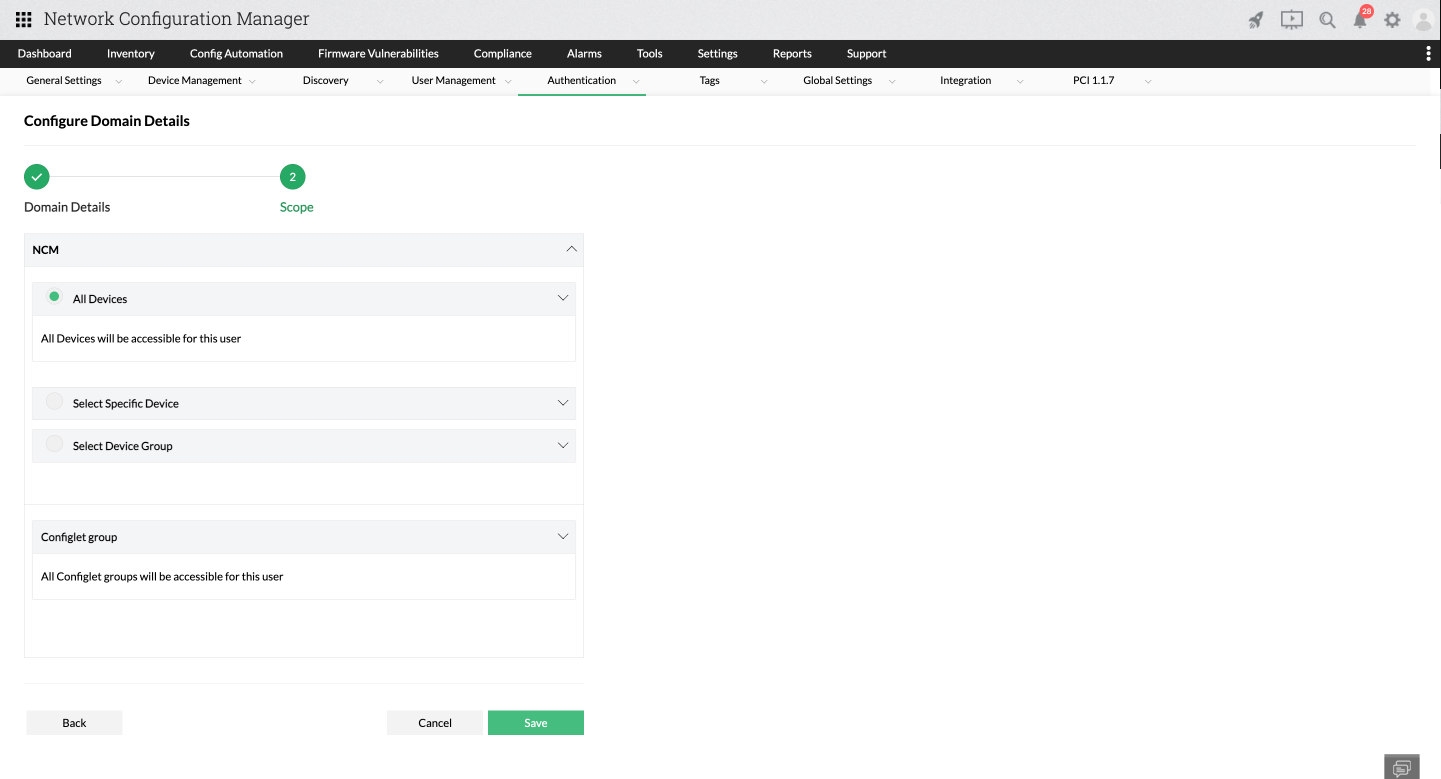This screenshot captures a webpage from the Network Configuration Manager. The interface is organized with a black border on the left side, containing a list of navigation options. From top to bottom, these options are: Dashboard, Inventory, Config, Automation, Firmware Vulnerabilities, Compliance, Alarms, Tools, Settings, Reports, and Support.

Beneath these primary options, there is a secondary set of options: General Settings, Device Management, Discovery, and User Management. Within this list, 'Authentication' is highlighted by an underline and a green line, indicating the current selection. Following 'Authentication' are additional options: Tags, Global Settings, Integration, and PCI or L, 1.1.7.

To the left of the main content area of the page, there's a header in dark text that reads "Configure Domain Details." Adjacent to this is a green circle with a white checkmark inside it. To the right, there is another green circle containing the number '2'. Below, a section labeled "Domain Details and Scope" appears, including a label 'NCM' encased in a text box-like designation. Underneath this is a circular icon with a green center labeled "All Devices," accompanied by text explaining that all devices will be accessible for this user.

Following this, there are unselected options for specifying device access: "Select Specific Device" and "Select Device Group." Further down, another option, "Configlet Group," states, "All Configlet Groups will be accessible for this user."

At the bottom of the page, there are two action buttons. The "Save" button stands out with its green background, positioned alongside the "Cancel" button.